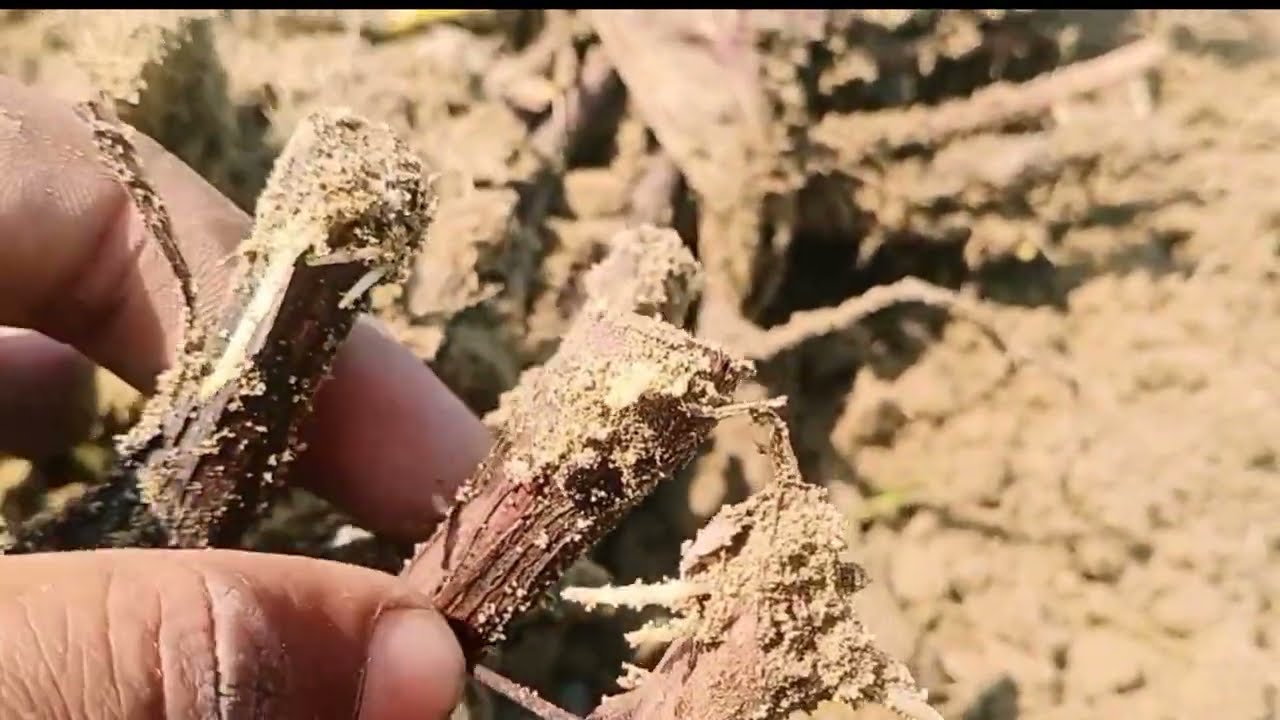The photograph captures a close-up view of an outdoor scene focused on a root structure held by a person's hand. Emerging from the left side of the image, the thumb and forefinger grasp a thick, woody root tangled with dirt and small granules of sand. In this close-up shot, the root consists of three connected segments, partially obscured by soil, and exhibits some new, lighter-colored growth sprouting out. The background, blurry but discernible as a muddy or dirt-covered area, shows scattered roots and sticks protruding from the ground. There are patches where the earth has been disturbed, possibly indicating recent digging or excavation activity. The overall impression is that of someone foraging or pulling up root vegetables or woody roots from a moist, textured landscape.